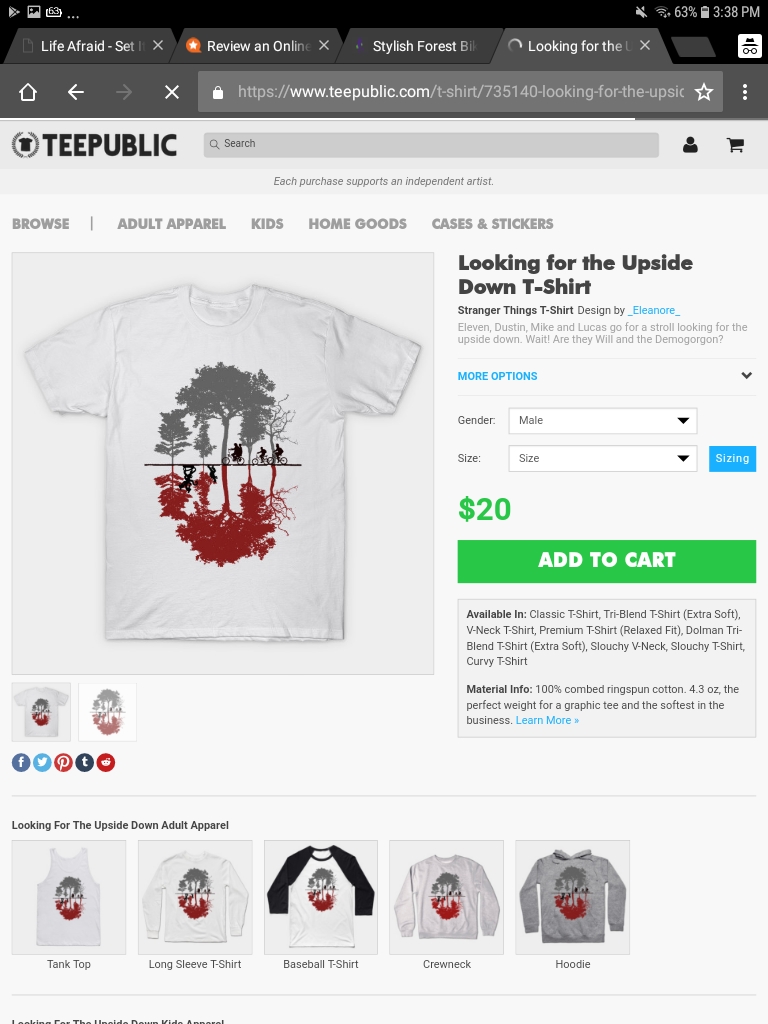The image is a screenshot of a website, likely taken from a phone due to the presence of the status bar at the top. The status bar displays several icons including the time, some logos, and a battery icon showing 63% charge. Below the status bar, there are tabs labeled "life," "afraid," "set review," and "online."

The website URL is visible and reads "https://www.tpublic.com/t-shirt/735140-looking-for-d-up," indicating this is a TPublic page viewed in Incognito mode (evident from the icon of a hat and glasses). At the top of the website, "TPublic" is displayed in bold letters. To the right, there are several icons: a search bar, a person icon, and a shopping cart.

Underneath this header, there is a navigation menu with options such as "Browse All," "Adult Apparel," "Kids," "Home Goods," "Case," and "Stickers."

The main content of the page features a white t-shirt with an artistic design. The upper portion of the t-shirt shows gray trees, while the lower portion mirrors this with red trees. There are also silhouettes of people riding bikes. This design is themed around "Stranger Things" and includes references to characters like Eleven, Dustin, Mike, and Lucas.

To the right of the t-shirt image, there is a description that reads, "Looking for the Upside Down T-shirt designed by Ellen Cree. Eleven, Dustin, Mike, and Lucas go for a stroll looking for the Upside Down. Wait, are they with Will and a Demogorgon?"

Below this, there's a section for selecting gender and size, including a drop-down menu and a blue sizing guide. The t-shirt is priced at $20 and has a prominent "Add to Cart" button. Additional options are available for materials and styles such as "Plastic T-shirt," "Tri-blend T-shirt," "Extra Soft V-neck," "Premium T-shirt," "Relaxed Fit Dolman," "Triblend T-shirt," "Extra Soft Slouchy V-neck," "Slouchy T-shirt," and "Curvy T-shirt."

Material information specifies that the t-shirt is made of 100% combed ring-spun cotton, weighing 4.3 oz. and described as the "perfect weight for a graphic tee" and "the softest in the business," with a "learn more" link.

At the bottom of the page, thumbnails show the same design available on different types of clothing, including a tank top, long-sleeve t-shirt, baseball t-shirt, and hoodie.